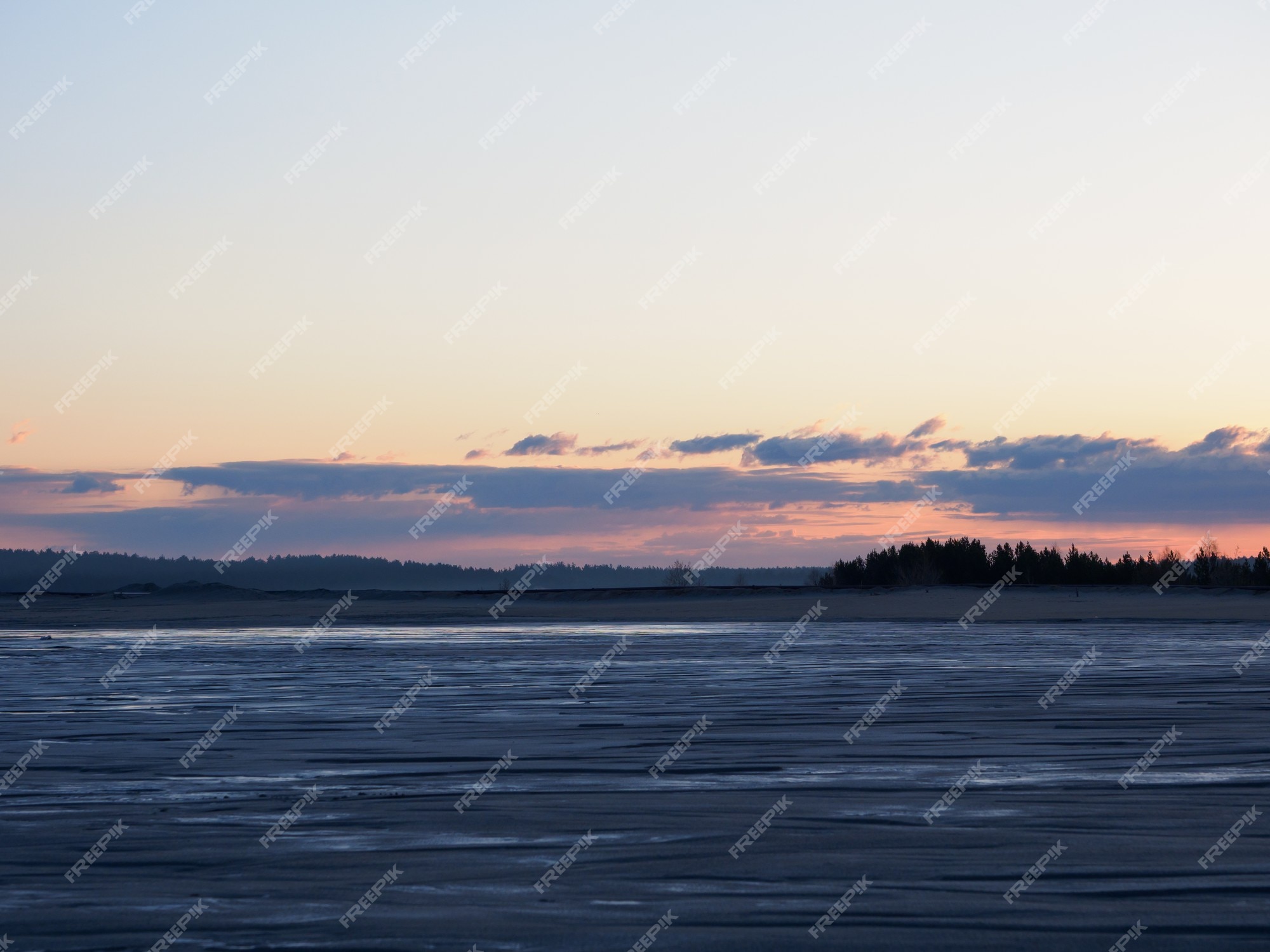The image captures a serene landscape at either dawn or dusk, featuring a calm river or lake in the foreground with gentle ripples on its surface. Along the bottom edge, a sandy beach is visible, leading up to a line of trees. Midway through the image, a road or bridge is discernible, adding an element of human presence amid the natural setting. The background reveals a dense forest with tree-lined hills, adding depth and a sense of wilderness. Above the horizon, the sky exhibits a warm salmon color, transitioning to a clear yellowish-gray tone as it ascends. Wispy, bluish-gray clouds hover near the horizon, complementary to the clear sky above. The scene is bathed in a soft orange glow, indicative of a sunrise or sunset, adding to the tranquil atmosphere. The image is marked with a watermark that reads "FREE PICK!" across its entirety.